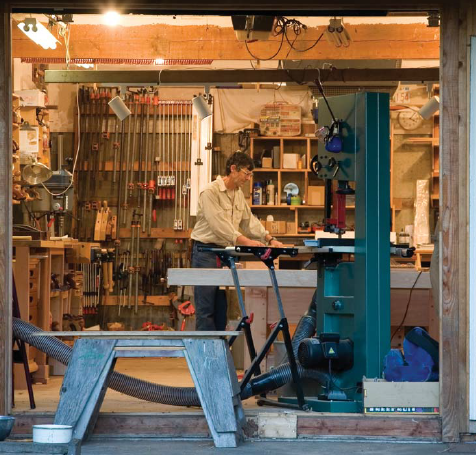In this photograph, a man is seen working diligently inside a well-organized workshop. The man, dressed in a beige long-sleeved shirt and blue jeans, has short black hair and wears glasses. He is positioned centrally in the image, facing toward the right and leaning over a surface, possibly feeding material through a saw or drill press. In the foreground, near the bottom left corner, there are two wooden sawhorses, one of which is supporting tools or materials. The workshop is notably clean and well-lit, with lighting coming from overhead, including fluorescent lights on the left side. The back wall of the shop is lined with bookcases and shelves filled with various tools and objects. On the right side, the shelves are designed with rectangular compartments each housing different sprays or tools. The left side features vertically arranged long tubular items. Additionally, some workstations and a bench with bowls can be seen towards the left side of the image. The photo appears to be taken from an outside perspective, looking into the orderly and well-lit workspace.